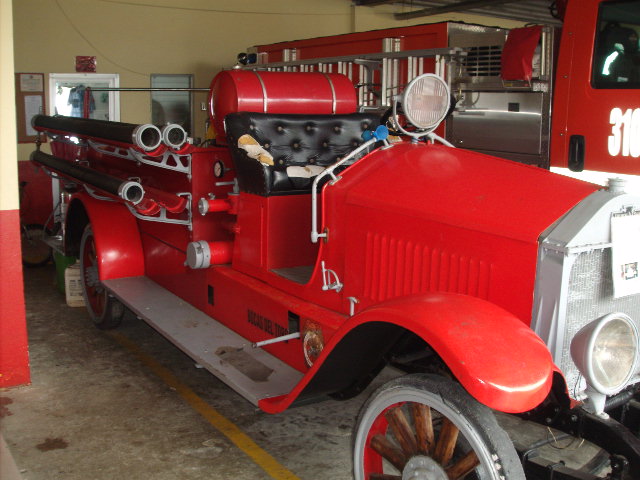The photograph captures the interior of a garage at a fire hall, featuring a juxtaposition of two fire vehicles. In the background, a modern, red fire truck with a metal ladder on the side stands out. In contrast, the foreground displays a vintage fire engine, styled in fire engine red with an open cab and black leather seating that shows signs of wear, particularly on the right-hand side. The wheels of the classic vehicle feature wooden spokes with thin rubber tires, reminiscent of early 20th-century design. This historic engine also boasts a single spotlight in front of the driver's wheel and carries long black pipes and red hoses on its back, suggesting its original firefighting purpose. The setting is a smooth, dusty concrete garage, with colored walls and a visible doorway, housing this fascinating mix of old and new fire apparatus.